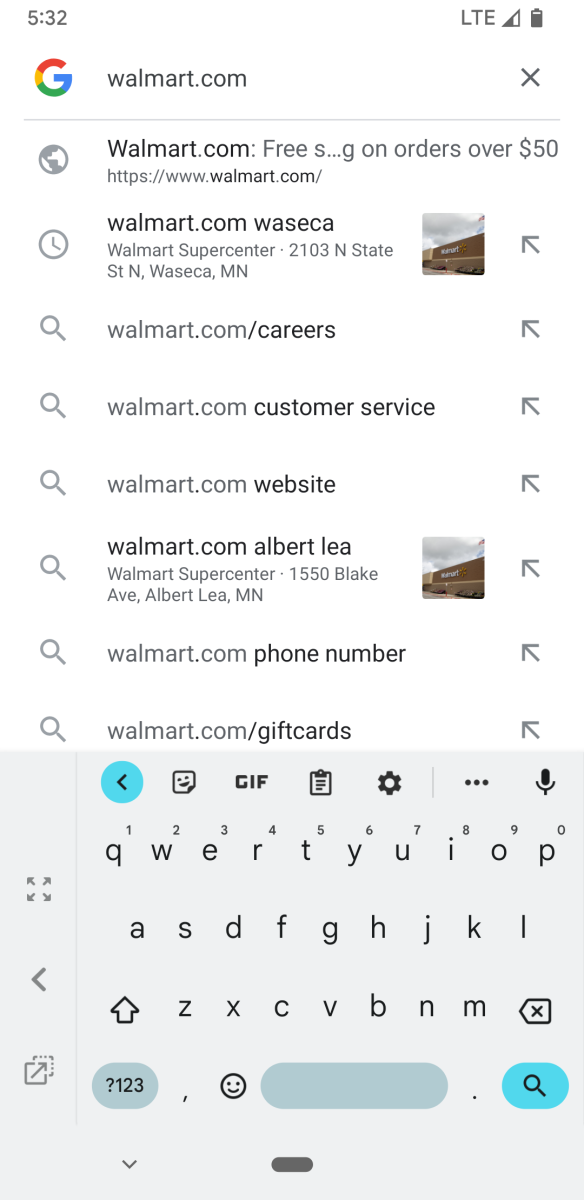In the screenshot of a Google search conducted on a mobile device, the details of the search results are meticulously captured. At the top of the screen, the time reads 5:32, and the device is connected to an LTE network with a signal strength of about half. The battery indicator shows that the battery is almost full. Below these indicators is the search query, "walmart.com."

The search results are as follows:
1. The first result marked with a globe icon, features "walmart.com" and the snippet "Free Shipping on orders over $50," followed by the URL "www.walmart.com."
2. The second result, indicated by a clock icon, reads "walmart.com" and mentions "Wasseka Walmart Supercentre, 2103 N State St, Wasseka, MN," with a small thumbnail image of a Walmart store.
3. The third result is for "walmart.com/careers."
4. The fourth result is for "walmart.com customer service."
5. The fifth result is "walmart.com website."
6. The sixth result points to "walmart.com Albert Lea Walmart Supercentre, 1550 Blake Avenue, Albert Lea, MN," accompanied by a thumbnail image that appears identical to the one for the Wasseka store.
7. The seventh result lists "walmart.com phone number."
8. The final result is for "walmart.com/gift cards."

At the bottom of the screen, the on-screen keyboard remains open, indicating that further searches can be initiated.